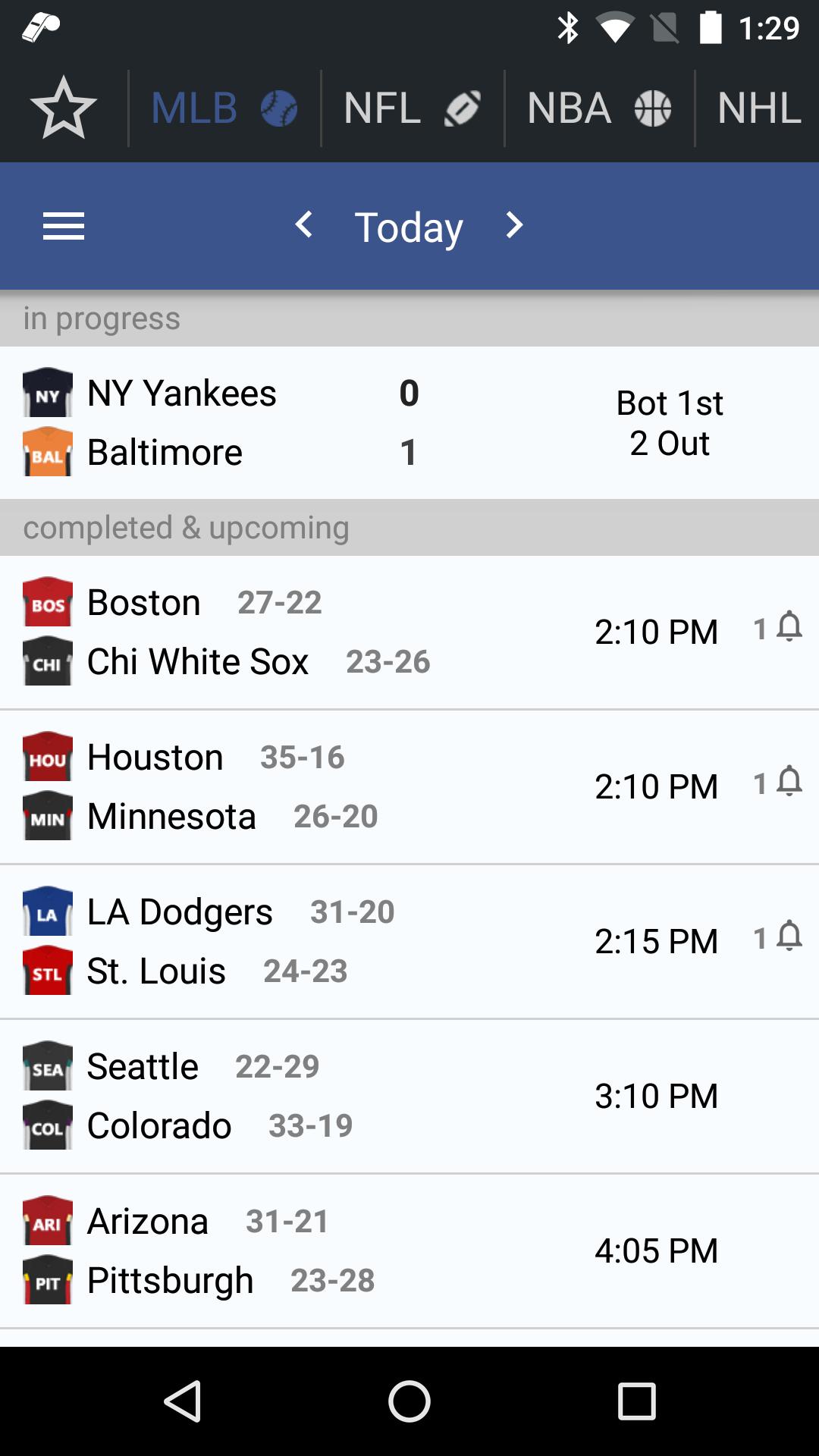This image showcases a sports app interface displaying the schedule and scores for Major League Baseball (MLB) games. The top black border of the screen features a white whistle icon in the upper left corner. On the upper right, icons for Bluetooth, Wi-Fi, a full battery indicator, and the current time (1:29) are visible.

Below this, a blue bar contains a horizontal three-line menu icon on the left and the currently active MLB section, indicated by a blue star icon and a baseball graphic. Other sports options such as NFL, NBA, and NHL are also listed but not currently selected.

The main part of the screen features the current and upcoming MLB games. At the top, under a "Today" header with backward and forward navigation arrows, the app shows an "In Progress" game: the New York Yankees versus the Baltimore Orioles, with a current score of 0-1 in the bottom of the first inning with two outs.

The "Upcoming" section follows listing the matchups, respective start times, and notification bell icons. The games include:
- Boston Red Sox vs. Chicago White Sox at 2:10 PM
- Houston Astros vs. Minnesota Twins at 2:10 PM
- Los Angeles Dodgers vs. St. Louis Cardinals at 2:15 PM
- Seattle Mariners vs. Colorado Rockies at 3:10 PM
- Arizona Diamondbacks vs. Pittsburgh Pirates at 4:05 PM

Each team name is accompanied by an image of a colored jersey to the left, providing a visual identifier for the teams.

Overall, this detailed breakdown captures all the vital elements and information presented on the sports app interface.